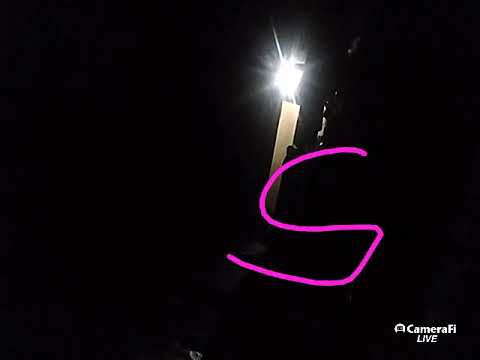The photograph captures a dark, nighttime setting dominated by black hues. Centrally, slightly off to the right, a brilliant white light illuminates the scene, casting its glow on a rectangular object situated directly beneath it. This object, displaying a yellowish tint, appears to be held by an indistinct figure or item. Superimposed on the image is a hand-drawn letter "S" in light purple, created with a crayon or digital pen, positioned towards the center-right of the frame. In the bottom right corner, white text that reads "Camera Fi Live" is clearly visible, accompanied by a small, indeterminate logo. The overall impression suggests a snapshot that's been digitally altered with artistic elements.